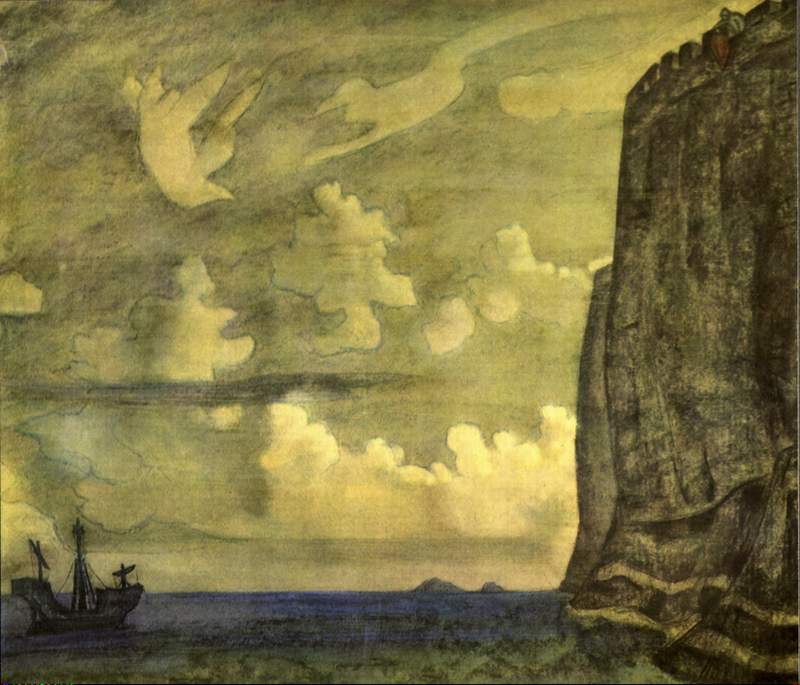The painting titled "Ambassador," also known as "Messenger Island," by Nicholas Roerich, created in 1914, presents a dramatic maritime scene. Dominated by a dark blue to light blue sea, the composition features a large ship with three masts, possibly a pirate or shrimp boat, sailing in the bottom left corner. Towering on the right side is a formidable cliff of stone, resembling an ancient or medieval fort with turrets reaching skyward. The earthy tones of the cliff blend seamlessly with the surrounding shrubbery and green grass at its base. The sky is a haunting mixture of olive green and gray hues, dotted with puffy white and yellowish clouds, adding to the painting's mystique. The entire scene is meticulously detailed with a symbolic and romantic style, combining elements of landscape, charcoal, and oil paint.